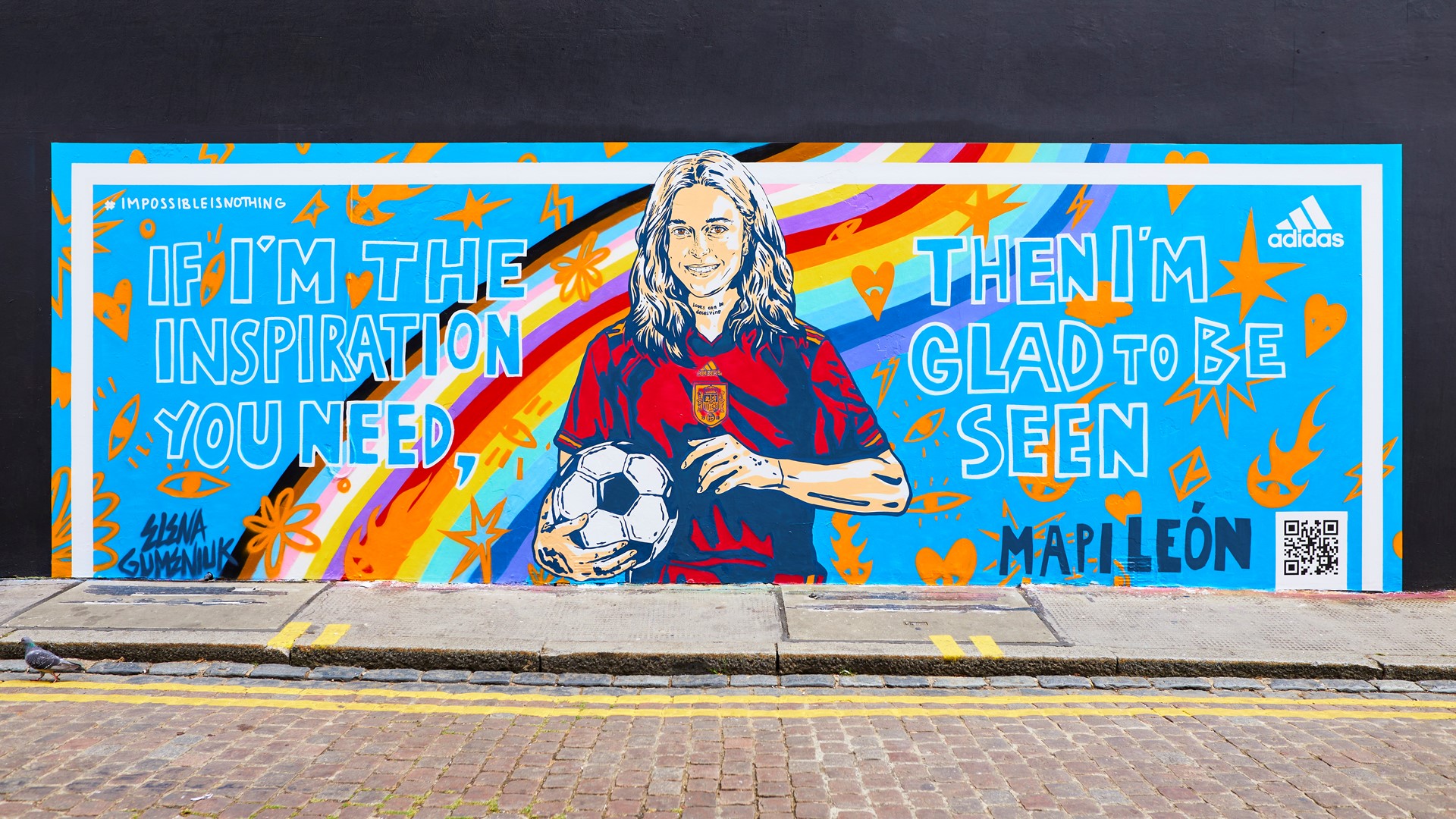The image features a street mural painted on a wall. The foreground includes a road made of worn-down red bricks with gray mortar between them, leading up to a curb. A double yellow line is painted in front of the curb, which steps up onto a concrete pedestrian walkway. The mural itself is rectangular with a predominantly blue background accented by a thick white stripe. The mural displays multiple lines of blue text with white borders that read, "If I'm the inspiration you need then I'm glad to be seen." In the bottom right corner, the artist's name, Mape Leon, is inscribed in blue text. The focal point of the mural is a painting of a woman dressed in a red uniform top, holding a soccer ball. Although the overarching color scheme is blue, there are hints of other colors suggesting a rainbow effect integrated into the background. This vivid and motivational mural acts as a large, horizontal sign facing the pedestrian walkway.